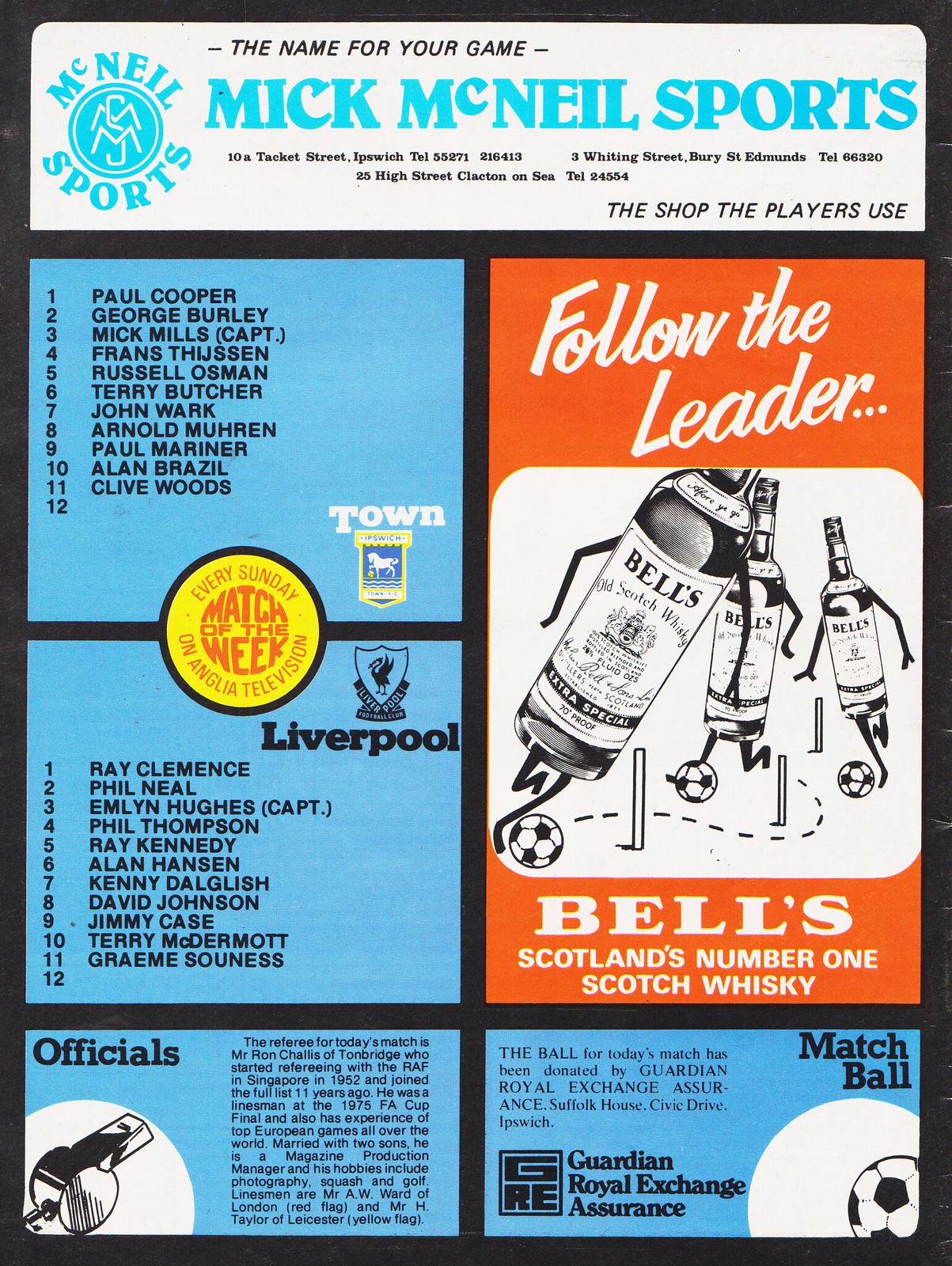The image appears to be the cover of a 1960s British soccer magazine with a black background, highlighted by a plethora of colorful advertisements. At the top, in a prominent white text box, it reads “McNeil Sports: The Name for Your Game,” followed by multiple shop addresses and telephone numbers: 10A Tackett Street, Ipswich, TEL 55271-216-4133; Whitting Street, Bury St. Edmunds, TEL 66320; and 25 High Street, Clacton-on-Sea, TEL 24554.

To the left side are two blue text boxes listing player names from 1 to 11, including notable figures such as Paul Cooper, George Burley, Russell Osmond, and Alan Brazil, with the 12th spot left blank. Adjacent to these, a red text box proclaims "Follow the Leader." Below, a playful illustration features three beer bottles labeled "Bell's Scotland's Number One Scotch Whiskey," seemingly engaged in a soccer match.

At the bottom right, another blue text box details the officials for the match: Ron Chalice of Tonbridge as the referee, highlighted for his extensive experience since 1952, including the 1975 FA Cup final. Linesmen listed are Mr. A.W. Ward of London (red flag) and Mr. H. Taylor of Leicester (yellow flag). Additionally, a blue text box mentions "The ball for today's match has been donated by Guardian Royal Exchange Assurance, Suffolk House, Civic Drive, Ipswich."

This intricately detailed cover merges professional soccer information with vibrant advertisements, encapsulating the essence of a classic sports magazine.